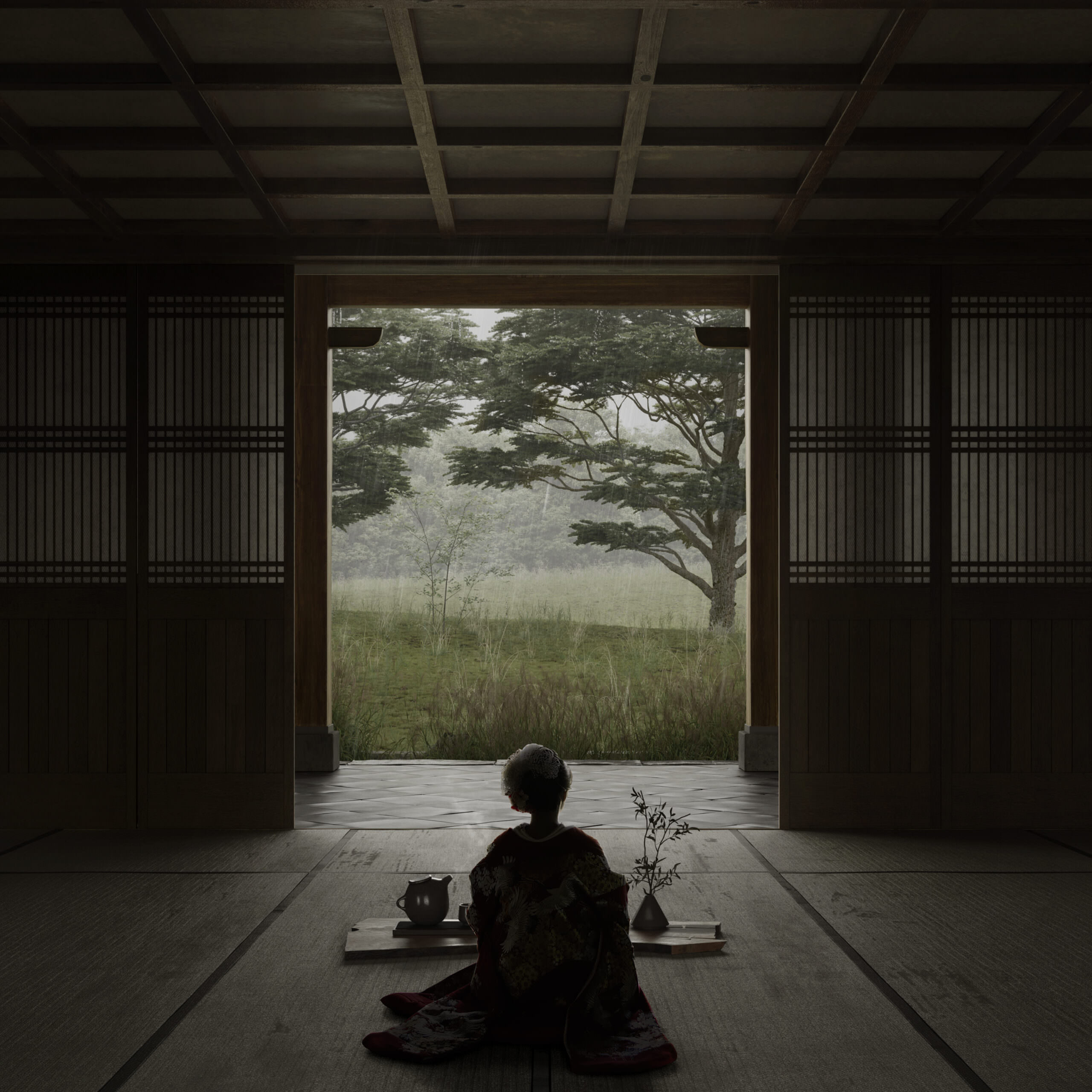The image exudes a serene and tranquil atmosphere, capturing a scene reminiscent of a Zen garden. Central to the composition is an open, square doorway that frames a lush green field with an array of verdant trees, complemented by distant hills and a wide tree to the right. Inside the room, which is cloaked in shadows and dominated by dark tones of black and gray, a woman in a floral kimono sits on the floor facing the open doorway. Her back is turned towards the viewer, adding a sense of contemplative solitude.

The flooring within the room appears grayish or dark, resembling traditional Japanese mats, with distinct black lines running across it. To the right of the woman, a vase with branches and leaves, perhaps part of an indoor plant, adds a natural element to the sparseness of the space. On her left side, a teapot or another vase is placed, contributing to the minimalistic aesthetic of the room. The surroundings include sliding doors typical of Japanese architecture, constructed with wood and paper.

The scene outside is illuminated by daylight, contrasting the dimly lit interior, and reveals tall grass and a paved or tiled area leading to two wooden columns. The overall mood is one of peaceful introspection, with the merging of indoor shadows and the soft outdoor light creating a cinematic and almost ethereal quality to the photograph.